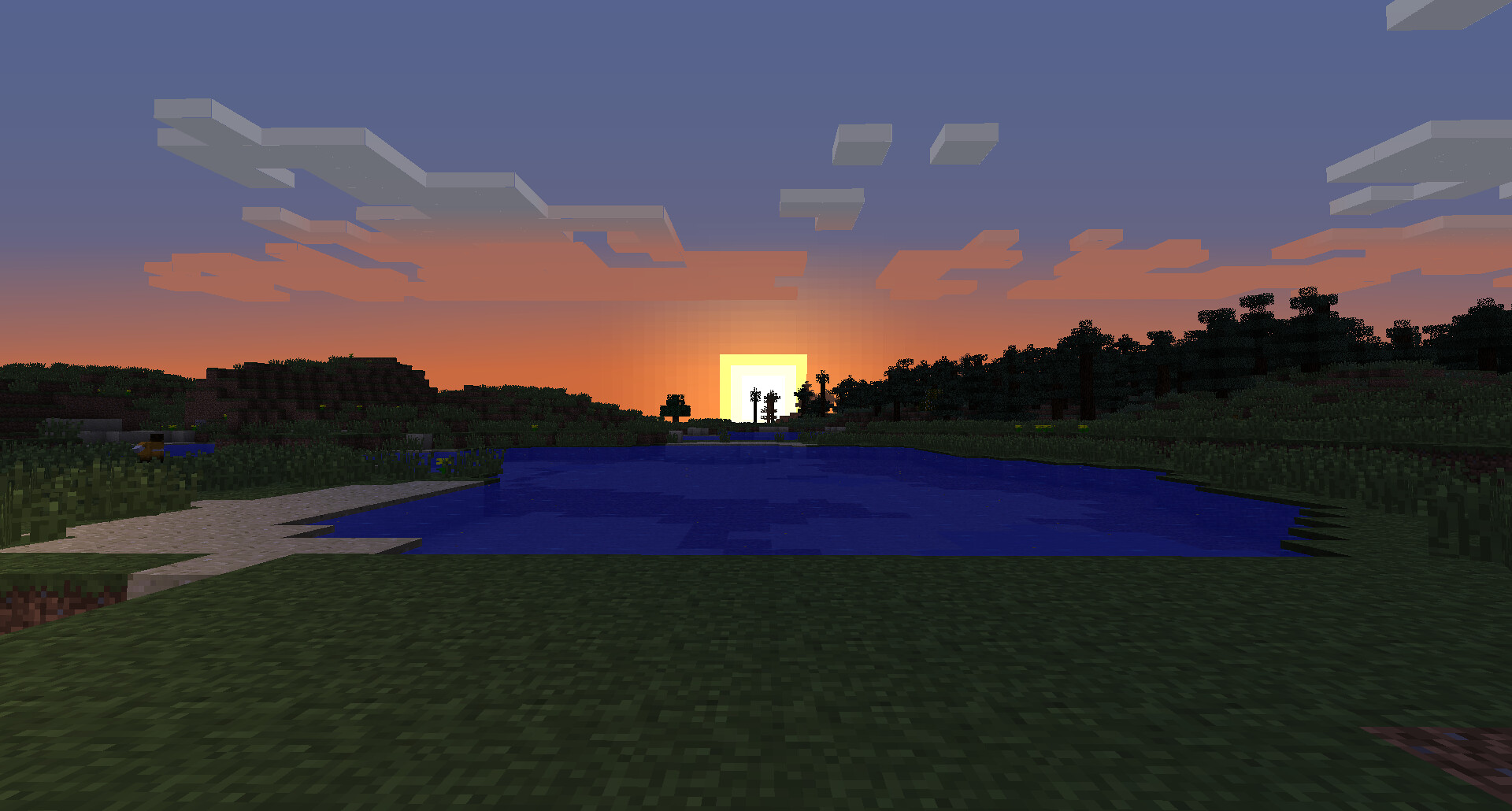The image depicts a computer-generated, Minecraft-like scene with a distinct, blocky aesthetic. Dominating the foreground is a vibrant green grassy field that transitions into a bright royal blue lake or pond, possibly representing a small body of water. On the left side of the lake, there are some bushes and a small stone walkway. As the landscape extends to the horizon, a tree line forms a dark silhouette against the striking sky, which captures either a sunrise or sunset. The sun appears as a bright yellow square with a thin outline of burnt orange above it, casting a warm, pinky-orange glow across the scene. Jagged, partly cloudy formations stretch out from the sun, transitioning from orange near the celestial object to white and then dark blue-purple as they reach the upper sky. Low hills and a few tree silhouettes, possibly palms, punctuate the background, enhancing the serene yet digitally stylized atmosphere of the scene.